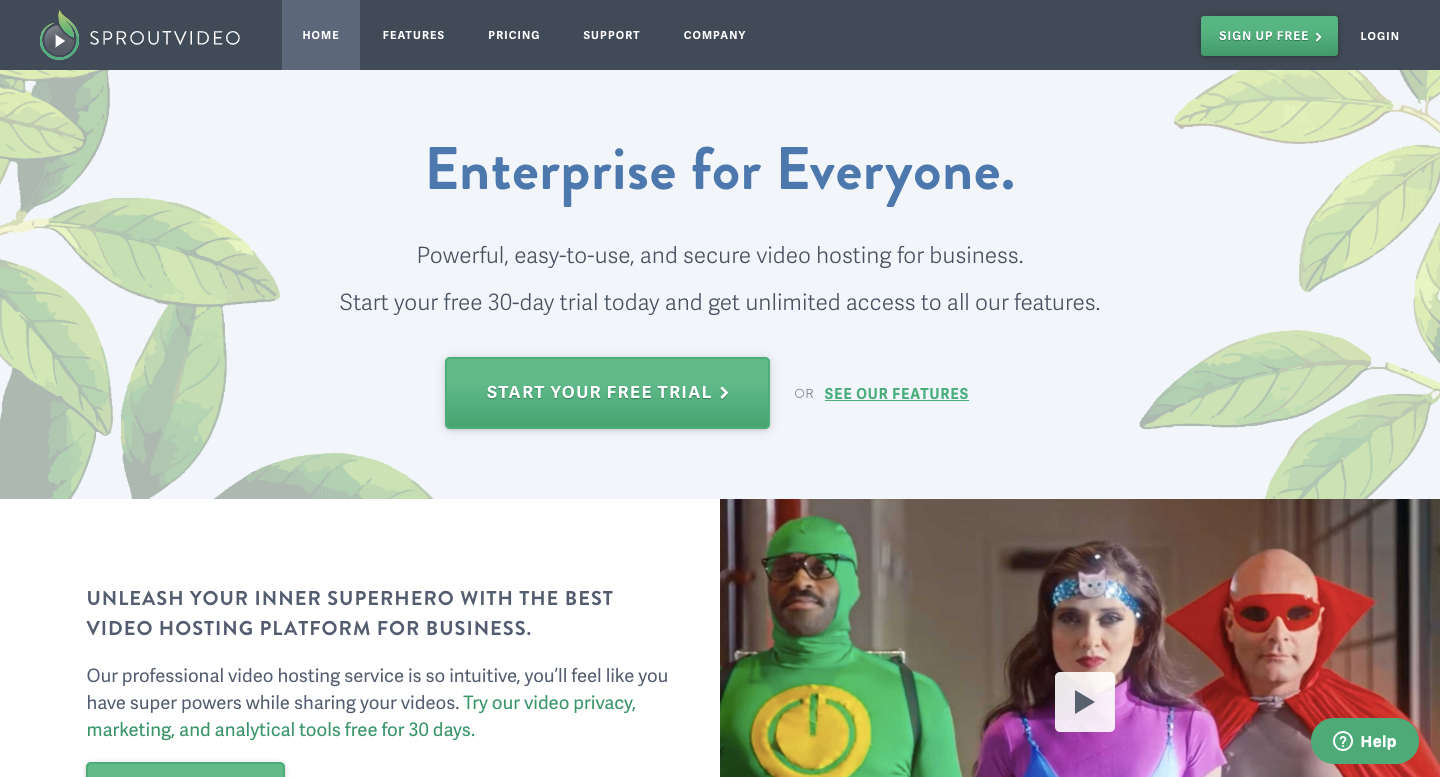The image depicts the homepage of a video hosting website, Sprout Video. The page is dominated by a gray and black header at the top, which features a green circular play button with a leaf attachment in the upper left corner, accompanied by the "Sprout Video" logo. The home button is highlighted with a gray square, indicating it has been selected.

Centrally positioned towards the upper part of the page is a gray rectangular banner adorned with leaves on both sides. Prominently displayed in the middle of this banner is a message that reads, "Enterprise for Everyone. Powerful, easy to use, and secure video hosting for business. Start your free 30-day trial today and get unlimited access to all our features." Below this message, there's a green button labeled "Start Your Free Trial," and to its right, a link that says "or see our features."

In the bottom left section of the page, there is a white text box area proclaiming, "Unleash your inner superhero with the best video hosting platform for business. Our professional video hosting service is so intuitive, you'll feel like you have superpowers while sharing your videos. Try our video privacy, marketing, and analytical tools free for 30 days."

On the bottom right, there is a graphic featuring three superhero characters. The figure on the left is a man in a green bodysuit with black eye markings, looking off to the left. The central figure is a woman with long dark hair and a headband featuring a cat emblem, dressed in a purple costume. The rightmost figure is a bald man clad in a red devil costume, including a red cape and a red mask. Embedding into this image is a play button in the form of a white square with a black triangle, indicating that there is a video available to watch. Lastly, in the bottom right corner of the page, there is a green oval button labeled "Help" which users can click for assistance.